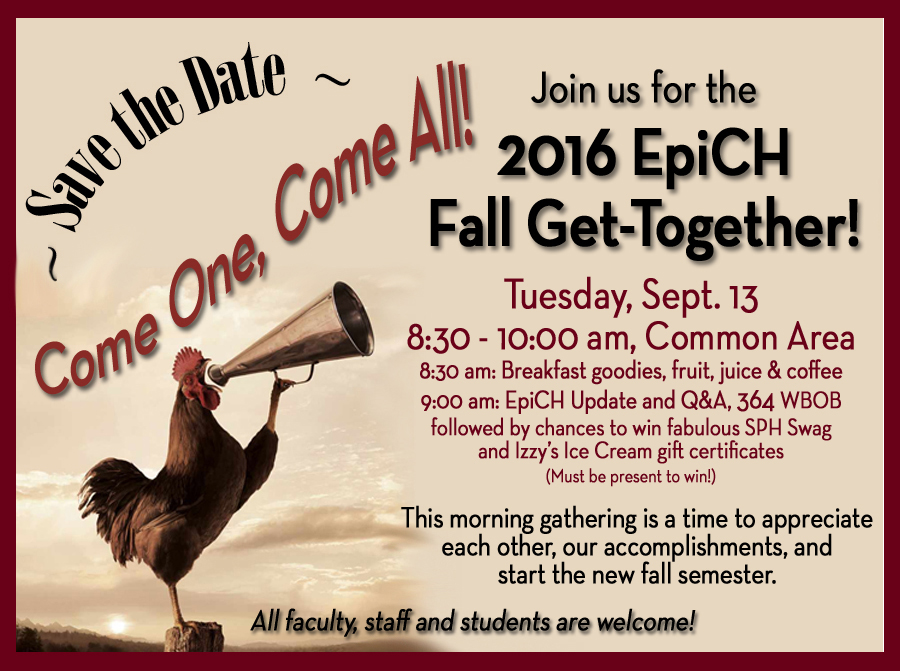Set against a tan background with a red border, this advertisement invites all faculty, staff, and students to save the date and attend the 2016 EPICH Fall Get Together. The event, which emphasizes community and the start of the new fall semester, is scheduled for Tuesday, September 13th, from 8:30 to 10:00 a.m. in the Common Area. At 8:30 a.m., attendees can enjoy breakfast goodies, fruit, juice, and coffee. This will be followed by an EPICH update and Q&A session at 9:00 a.m., hosted by 3.64 WBOB. Participants will also have the chance to win fabulous SPH swag and Izzy's ice cream gift certificates, provided they are present to win. The flyer features a prominent image of a rooster using a megaphone on the left side, adding a whimsical touch to the announcement. The message "Come one, come all!" invites everyone to join in the celebration and appreciate each other's accomplishments.